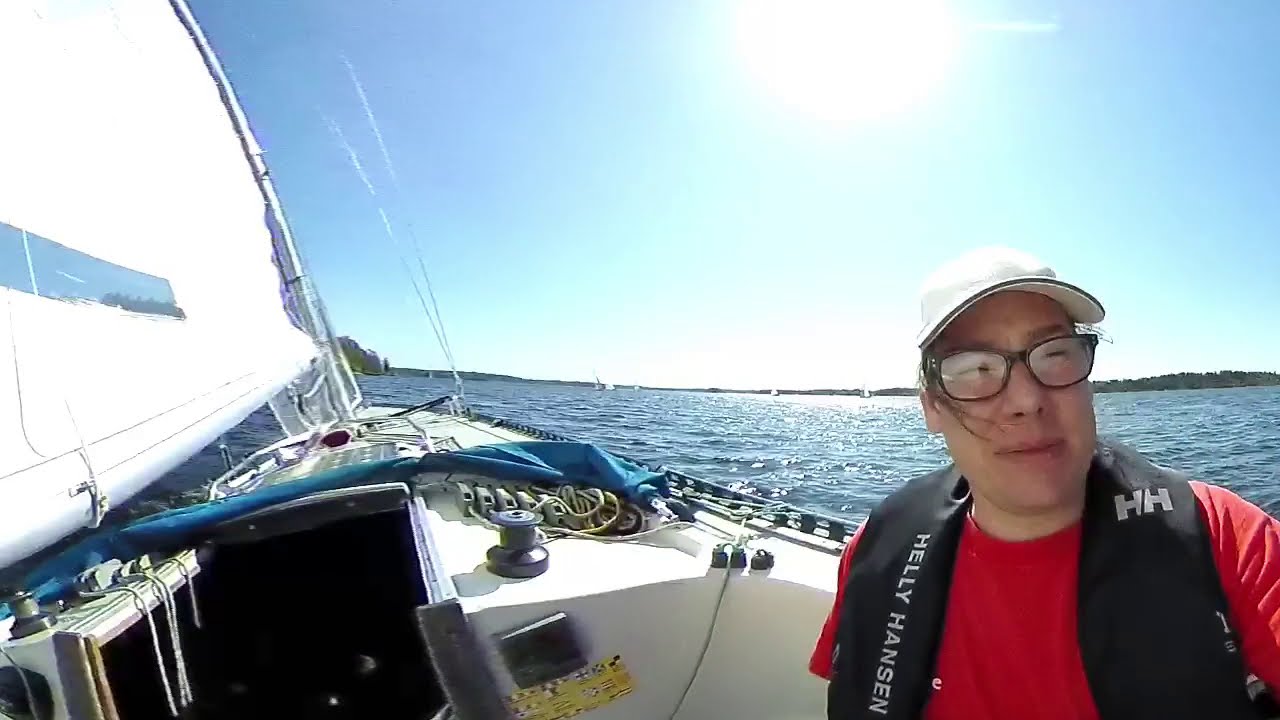The image captures a vibrant scene of a person standing on the deck of a large, modern white sailboat, taking a selfie. The individual, who appears to be Asian, has long hair and is wearing a white baseball cap, glasses, a red t-shirt, and a black safety vest with the brand "Helly Hansen" visible on it. The sailboat rocks slightly in the calm waters, displaying various fittings, ropes, and a blue rolled-up tarp. A tall, white sail stands prominently in the background. The water below reflects the bright sunlight of a clear, sunny day, with small, gentle waves visible on the surface. In the distant background, some tree-covered hills or islands can be seen on the horizon. The sky above is a vivid blue, devoid of clouds, with the sun shining brightly, adding to the warm and sunny ambiance of the scene.